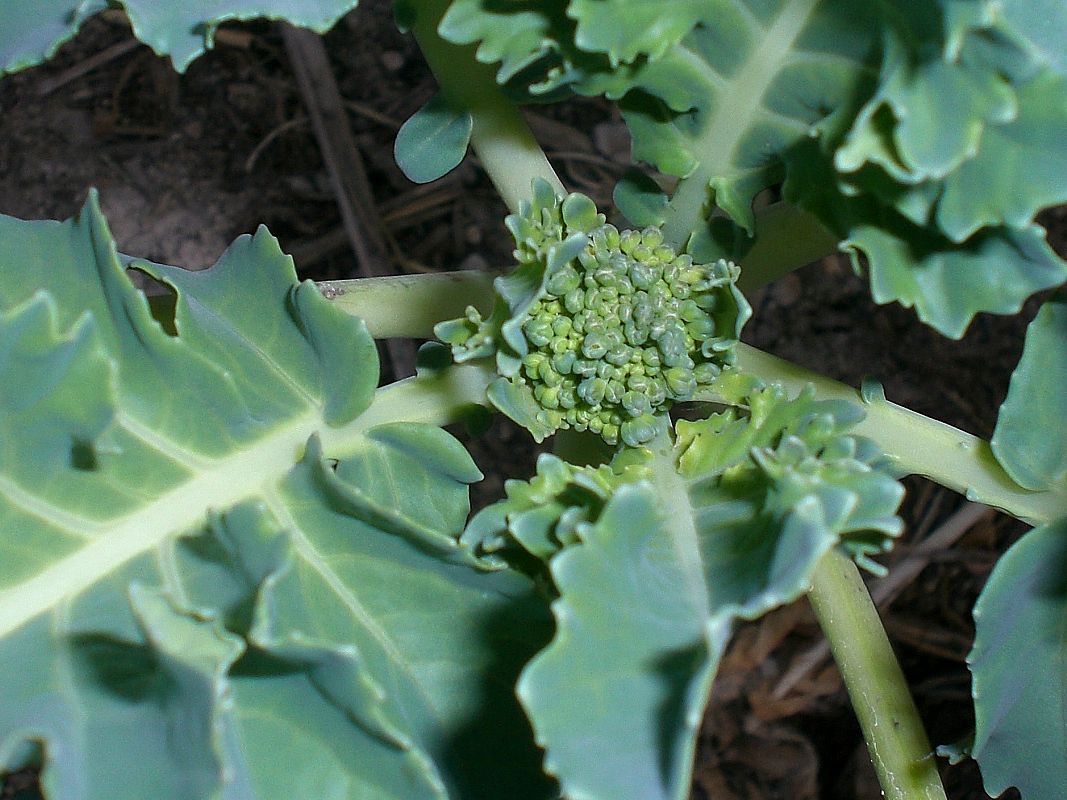This close-up, top-down photograph captures a dark green plant with its intricate details vividly. The plant features robust, light green stems that radiate outward, forming a star-like pattern with two stems extending diagonally upwards, two to the sides, and two downward. These stems support large, shiny green leaves, which appear almost plastic-like due to their glossiness. The plant is rooted in chocolate-brown soil, interspersed with sticks and the branches of neighboring dark green plants. At the core of the plant lies a dense cluster of small lime-green buds or seeds, resembling tiny beans, which are tightly packed and flanked by dark green leaves. These central buds vary in size, with some reaching the size of peas, creating a beady texture in the plant's heart. The photograph offers no definitive clues as to whether these central structures are flower buds or seeds.